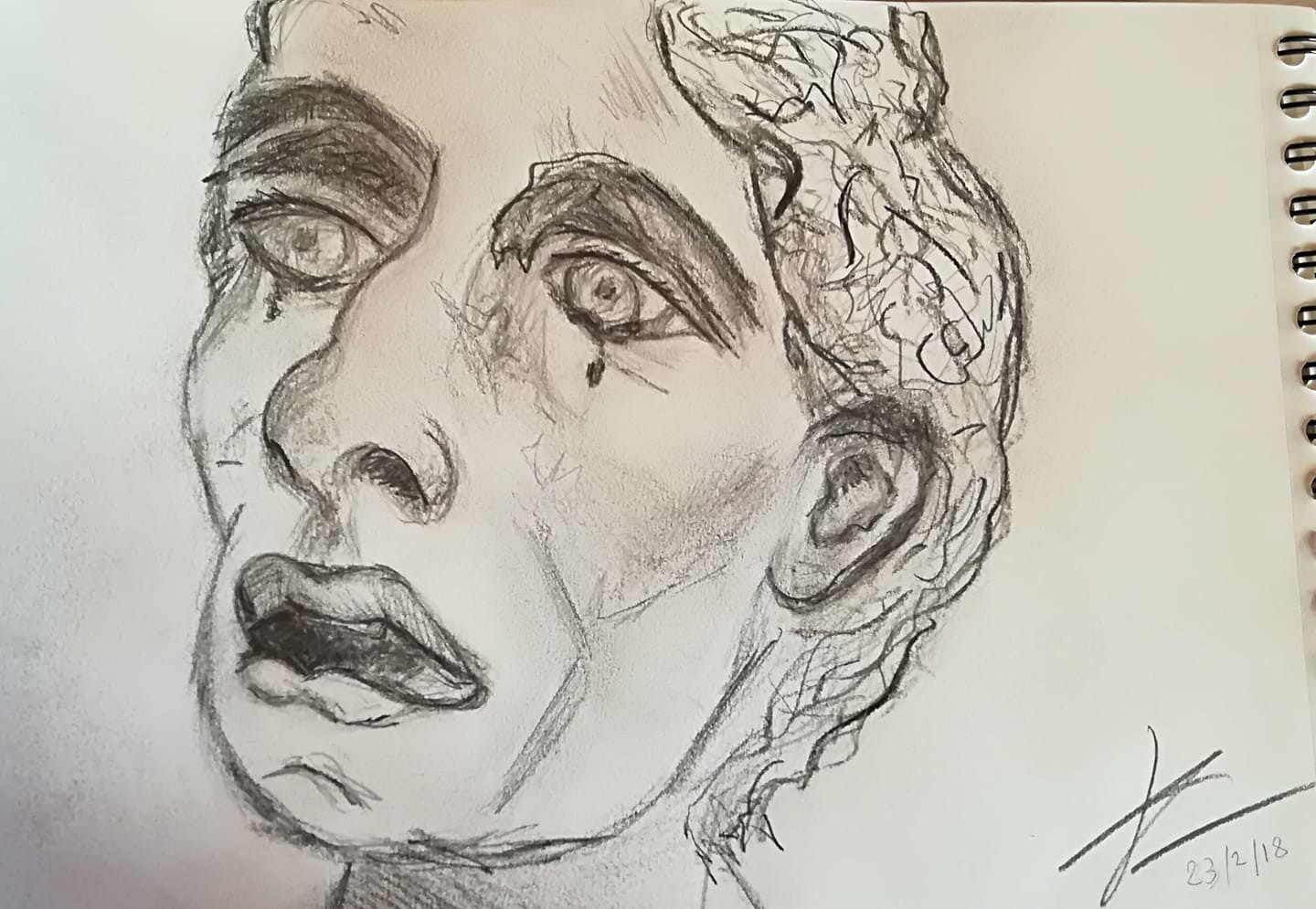This is a detailed close-up photograph taken indoors, capturing a piece of artwork inside an art notebook. The black spiraled binding runs vertically down the right side of the image. In the bottom right corner of the page, there is a signature along with a date, which appears to be February 23rd, 2018. The artwork is rendered entirely in pencil, depicting the head of a person with short hair, potentially male, gazing to the left. The figure has large, bushy eyebrows, prominent eyes with visible tears streaming down from each, a relatively big nose, and a slightly open mouth, conveying a profound sense of sorrow.